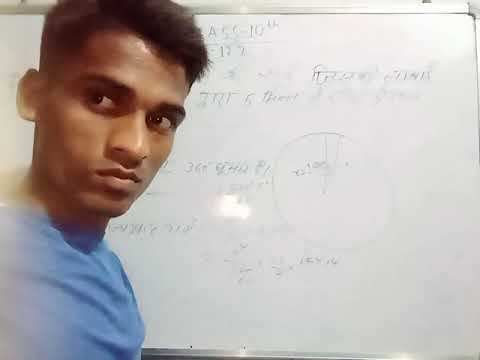The image depicts a young Indian man with short brown hair, wearing a blue t-shirt, positioned on the left side of the frame. He has a blank, somewhat stern expression, with his eyes sharply looking to the left. Behind him, there's a whiteboard bordered in silver that is filled with various mathematical equations and a large pie chart with a small segment missing. While the equations are blurry and hard to read, one part at the top is discernible, showing "AS5 equals 1 0" and "a tenth over 12 7." The scene suggests he might be teaching or recording a video, possibly for an educational purpose such as a college or high school math lesson. He appears to be showcasing his work on the whiteboard.